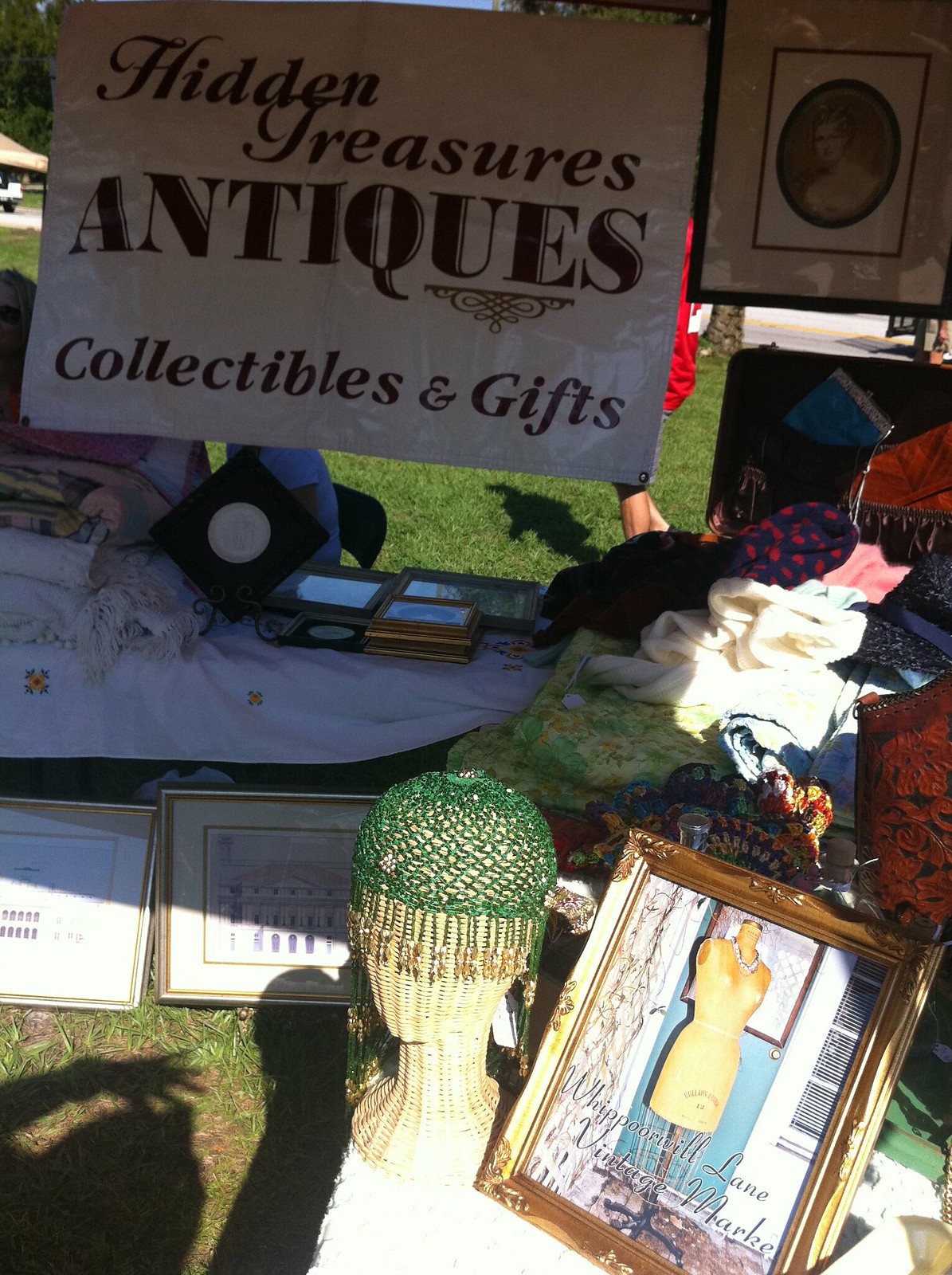The photograph, captured in full color during daylight, depicts an outdoor scene illuminated by sunlight, casting noticeable shadows. Situated on grass, the setting appears to be an arts and crafts type festival, specifically focused on hidden treasures, antiques, collectibles, and gifts. The image showcases various items arranged on the ground, including indistinct articles that could be clothing or pictures. Prominently, there is a mannequin head adorned with a gray, crocheted cap embellished with tassels and beads. Nearby lies a framed photograph of a tailor's mannequin, adding to the vintage theme of the display. A notable sign made of fabric is visible, inscribed with "Hidden Treasures, Antiques, Collectibles, and Gifts" in brown lettering on a white background. Additionally, there is an old framed picture of a woman and various other items like old clothes or blankets on the table, further enhancing the nostalgic ambiance of the stall set in what seems to be an outdoor market or fair.